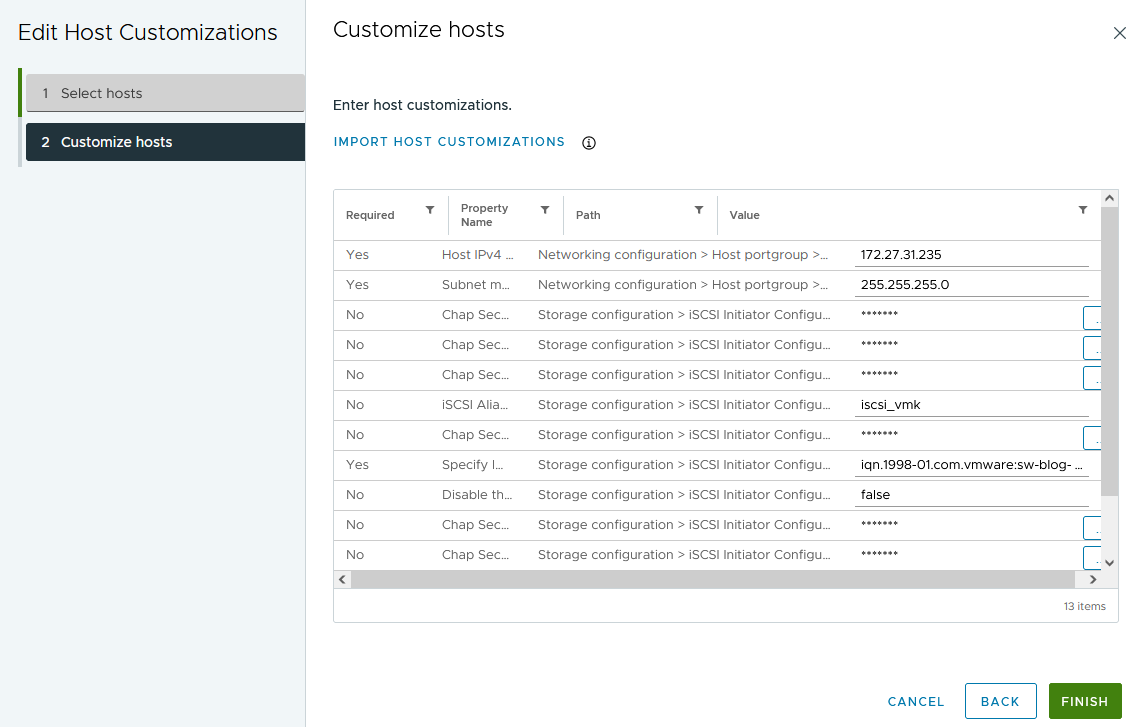The image appears to be a screenshot from a computer interface with two main sections. 

**Left Section:**
- A gray sidebar titled "Edit Host Customizations."
- It contains two options:
  - The first option, "Select Hosts," is within a gray border.
  - The second option, "Customize Hosts," is highlighted with a black underline.

**Right Section:**
- A white main area titled "Customize Hosts" in the top left corner.
- Directly below, there's a subtitle, "Enter Host Customizations."
- Further down, a blue heading reads "Import Host Customizations," followed by a detailed chart.
  - The chart has four columns labeled:
    - "Required" (entries appear to be either 'yes' or 'no'),
    - "Property Name,"
    - "Path,"
    - "Value"
  - Some entries in the "Value" column have numbers filled in.
- A gray scroll bar is located on the right (vertical) and at the bottom (horizontal) for navigation.